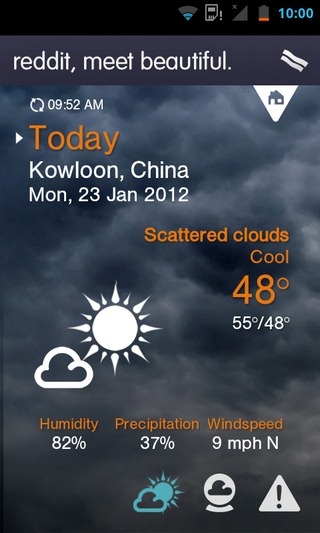A screenshot taken from a mobile phone at 10 o'clock shows a low battery and no cell service, potentially due to a missing SIM card, though the device is connected to the internet. The top bar displays the Reddit header "Meet Beautiful" with a couple of wave icons to the right. Below this, a refresh bar indicates "9:52 AM" along with home and dropdown icons. 

The main section of the screen provides detailed weather information for Kowloon, China on Monday, January 23, 2012. The forecast notes scattered clouds and cool conditions with a temperature of 48°F, a high of 55°F, and a low of 48°F. The humidity stands at 82%, with a precipitation chance of 37%, and a northerly wind speed of 9 mph. 

Visual icons towards the bottom include an overcast cloud symbol, indicating cloudy conditions, followed by a second icon displaying a cloud within a circle, possibly depicting more detailed weather data, and lastly, a triangle with an exclamation point, signaling a weather warning. The background of the weather section is a dark gray overcast, complementing the forecast.